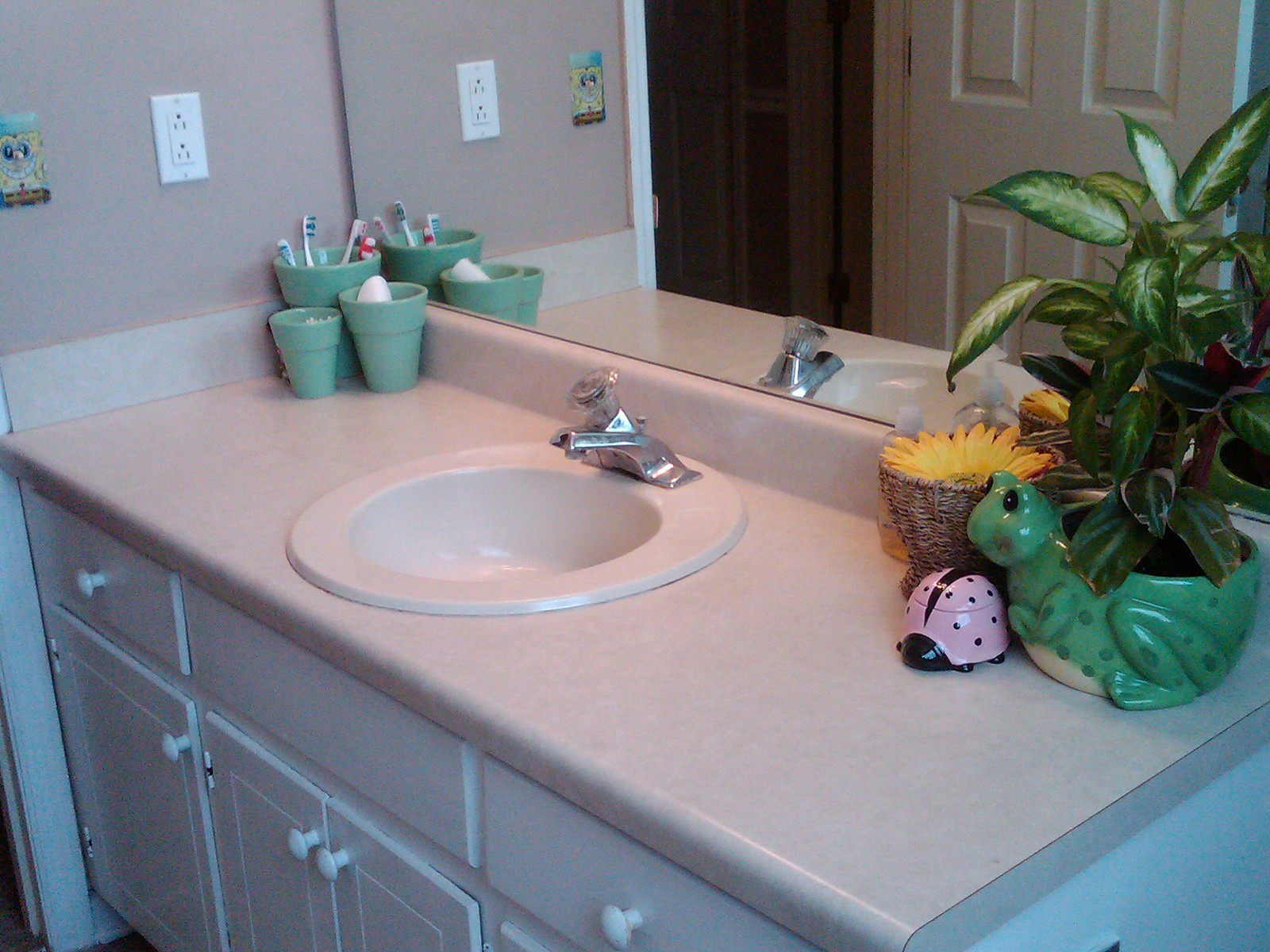In a cozy bathroom illuminated by soft lighting, the back left corner features a pristine gray and white power outlet. Adjacent to it on the right is a gleaming mirror that reflects an open wooden door, adorned with a four-paneled square design, revealing a hallway beyond. The laminate countertop beneath is a touch of practicality, adorned with three light green cups neatly placed in the corner. The far left cup holds two brushes, while the other cups partially obscure some indiscernible items. To the right of the cups is a modern sink with a sleek silver faucet, accompanied by a twist-handled silver candle holder beside it. 

On the extreme right, a charming woven basket brims with vibrant yellow flowers, accented by a decorative purple ladybug with distinctive dots. Nearby, a flower vase painted green with dotted patterns and sprouting lush green leaves adds a fresh touch of nature. Below, a few drawers with sturdy handles are slightly open, hinting at the room's inviting blend of functionality and homestyle charm.